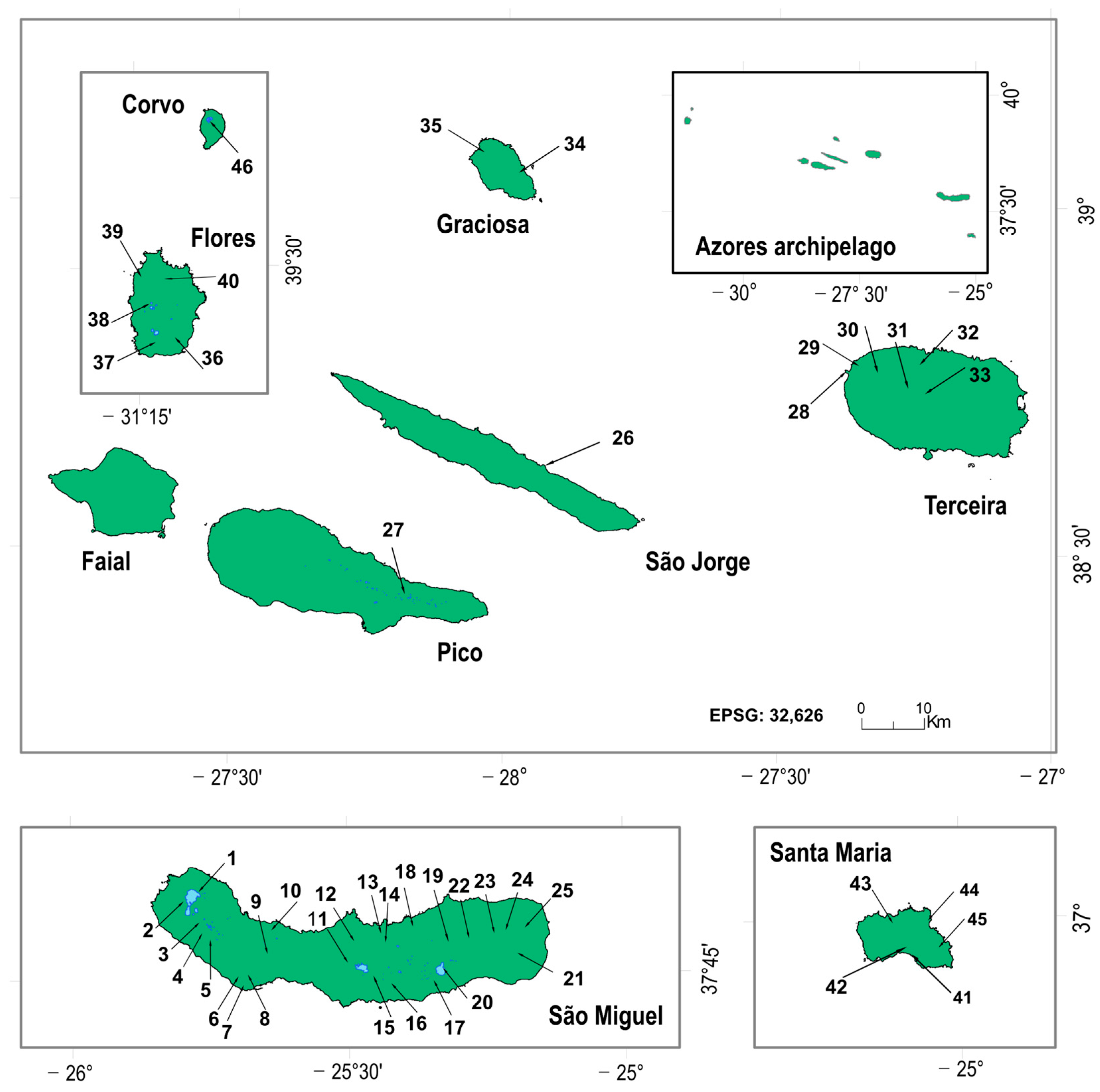This image is a detailed illustration of multiple maps, segmented into three distinct fields, each rectangular in shape, with the largest one positioned at the top. The top map prominently features various green-colored landmasses with labels in a foreign language, such as "Azores, Arquipelago," "Pico," "Sao Jorge," "Terceira," and "Graciosa." This section includes intricate details like numerous numerical labels indicating degrees and unspecified measurements, with figures ranging from -31 to 39 degrees. Additionally, there are smaller inset rectangles within this larger top map, showcasing places like “Corvo," and "Flores," with corresponding numerical data.

Beneath the top map, there are two smaller rectangles. The first, labeled as "Sao Miguel," spans from 1 to 25 in numeric values, accompanied by degree indicators varying from -26 to 30. Adjacent to this, a smaller, square map labeled "Santa Maria" displays measurements running from 41 to 45 degrees, indicating a temperature range from -25 to 37 degrees. Each map is detailed with lines connecting various points, illustrating specific spots and degrees, although the exact nature of these numbers remains unspecified. The overall color scheme features green landmasses against a backdrop of labeled measurements and degrees, providing a rich, detailed geographical representation.